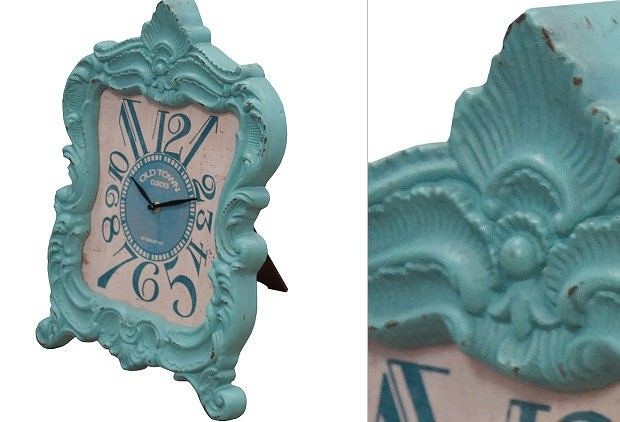The image is split into two sections, with two photographs displayed side by side. On the left, there is an ornate clock encased in an elegant, light blue, picture frame-like design. The frame is intricately curved, evoking the appearance of a mirror frame with its sophisticated style. The clock itself has a white face adorned with uniquely styled, light blue numbers. The corner numbers are notably larger, while the numbers near the top and sides vary in size, creating an interesting and visually appealing pattern. The clock hands are small and black, contrasting sharply against the white background. At the center of the clock face, the words "Old Town Clocks" are prominently displayed.

To the right, a zoomed-in photograph showcases a detailed view of the top portion of the clock. This close-up highlights a seashell-like design, crowned with a small, spherical ornament. Both the intricate design and the sphere maintain the same light blue hue as the frame, emphasizing the clock's cohesive and elegant aesthetic.